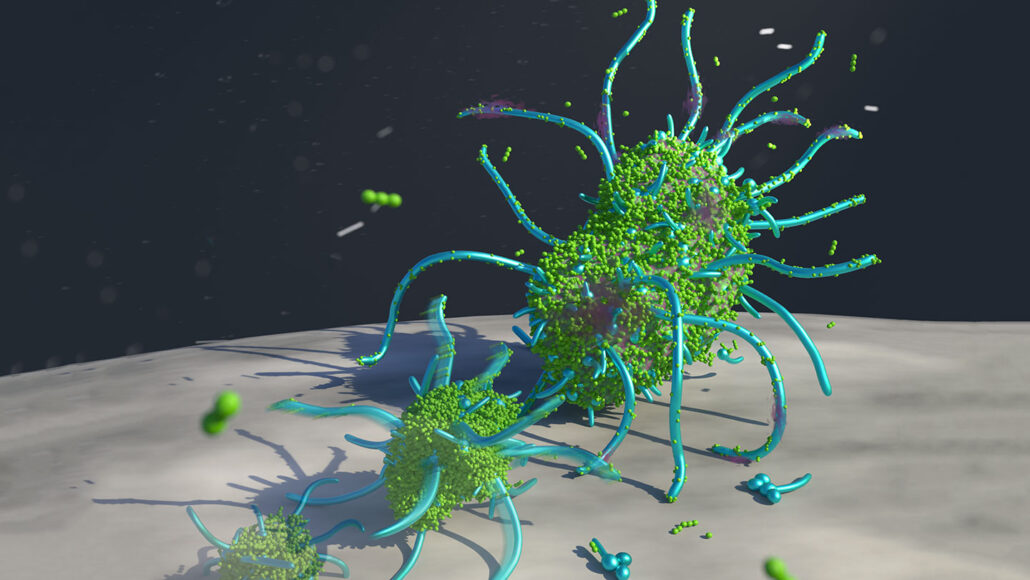The image appears to be a computer-generated animation or an enlarged microscopic view, depicting a scene with green, oval-shaped bacterial cells that possess numerous slender blue tentacles. These cells are positioned on a flat, gray surface that resembles the texture and color of the moon, set against a completely black background with a few scattered specks. The bacterial cells seem to be composed of many smaller spheres, and there are fragments of green and blue, likely detached pieces, floating or lying around the main subjects. The composition arranges these cells from back to front in a progression of sizes, from a huge cell to a smaller one, followed by an even smaller one in the foreground.